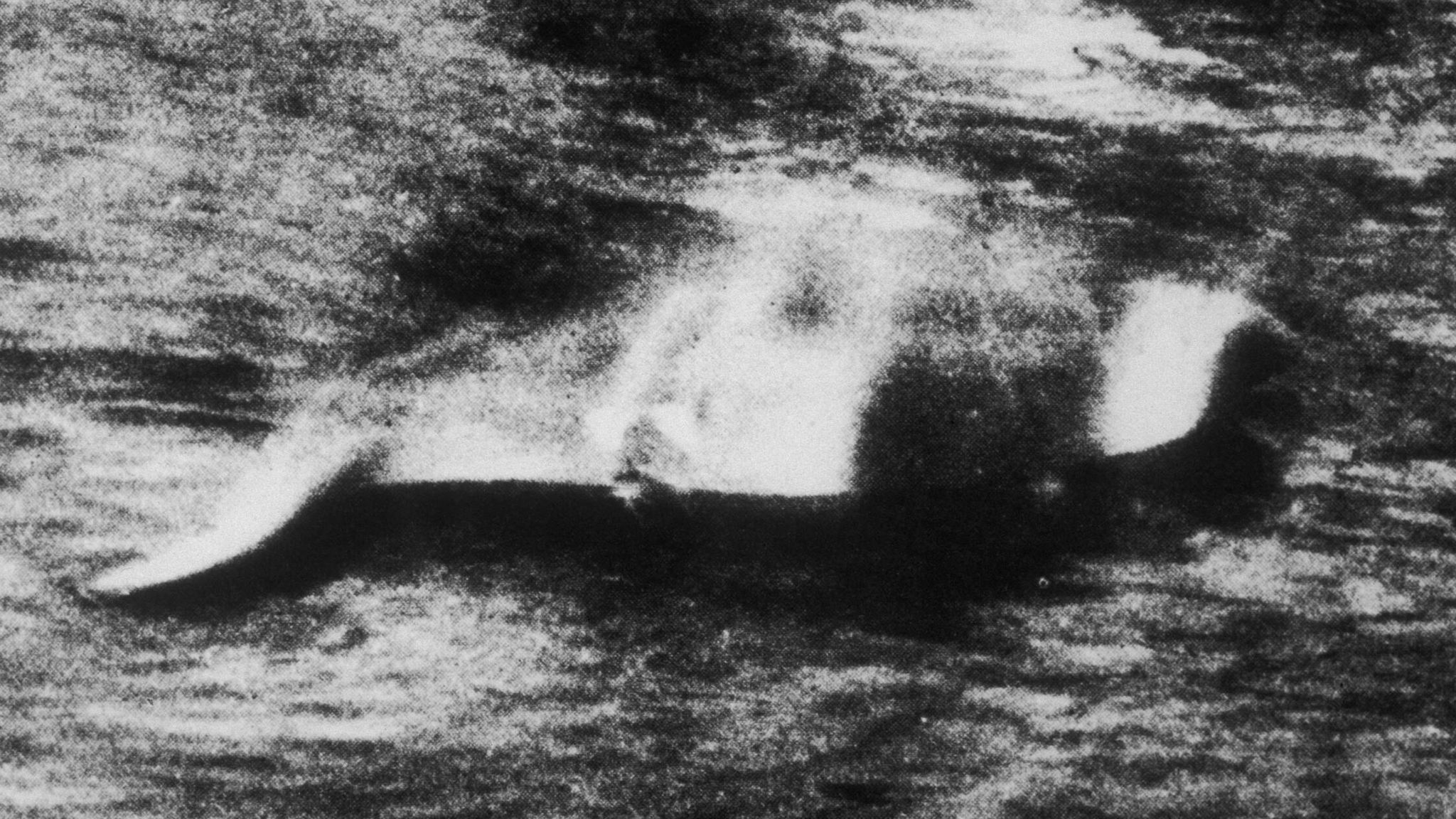This black and white photograph appears to be a low-quality, heavily pixelated and blurry image, resembling the kind of questionable photos often associated with mysterious or hoax phenomena like the Loch Ness Monster. The image, presented in landscape orientation, is characterized by a mix of dark and light streaks, creating an overall fuzzy and hard-to-read appearance. At the center of the photograph, there is a dark shape that is difficult to identify; it could resemble something serpentine, a fish, or even a boat with indistinct figures possibly sitting inside. The unclear outlines may also suggest the profile of a large marine creature, like a whale, swimming in choppy, rough seas with visible white caps. Despite the various interpretations, the image's quality and details remain too poor to conclusively determine the subject, lending itself to the air of mystery and speculation.